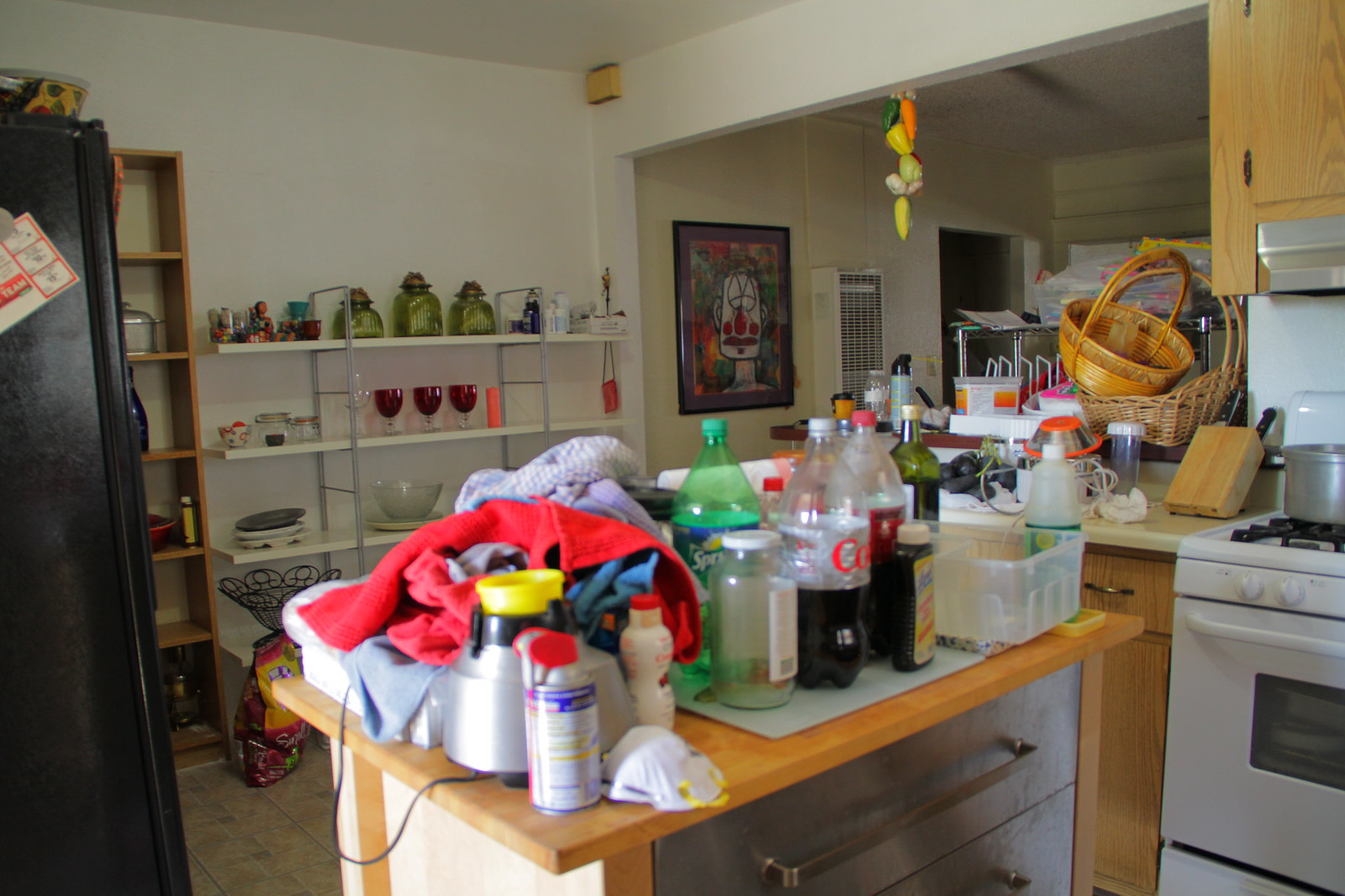In this image, we see a bustling and somewhat disorganized kitchen. The focal point is a central island with a wooden finish and metallic doors, cluttered with a variety of items. Prominently displayed on the island are several bottles, including a Coke bottle, a Sprite bottle, and others. Scattered across the island are also various other items, such as a box of Honey Bunches of Oats and some clothing.

In the background, there are shelves painted white, holding an assortment of glassware in different colors, including green and red pieces. The left side of the image features a large black refrigerator. Two wicker baskets can be seen in the distance, adding to the eclectic mix of textures and materials in the room. Overall, the kitchen has a lived-in and somewhat untidy appearance, lacking in organization but rich with details and everyday objects.